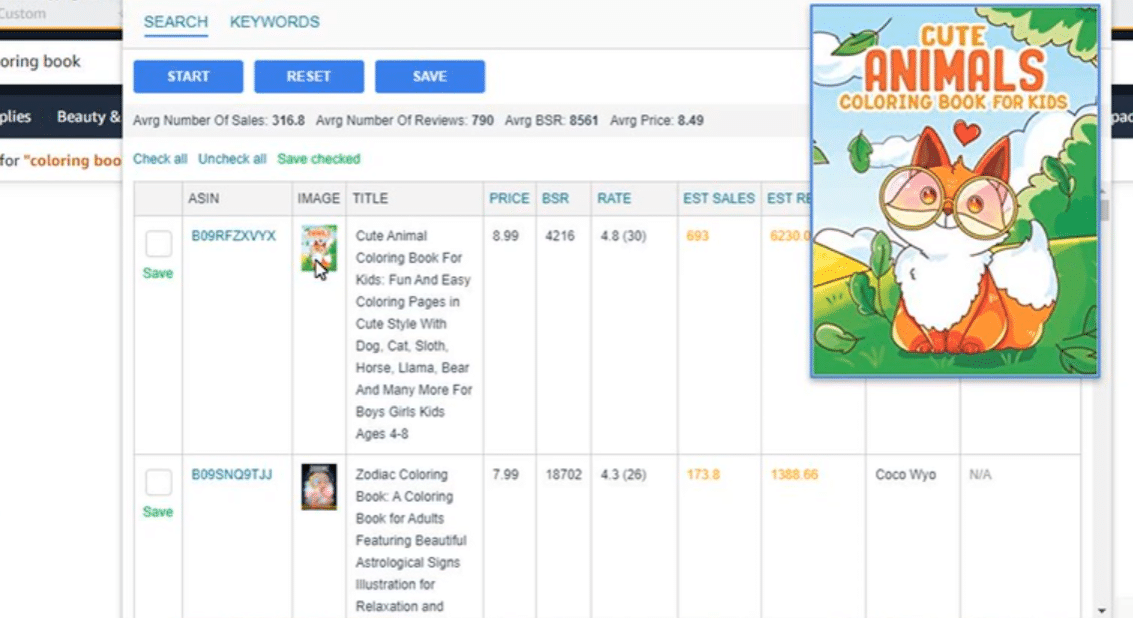**Image Description:**

At the top of the image, there is a light gray header. To the left side of the header are two tabs with blue, capitalized lettering. The first tab, labeled "SEARCH," is selected, indicated by a bold blue line underneath it. The second tab is labeled "KEYWORDS." 

Below the header, there is a gray line divider, followed by three rectangular buttons with rounded edges. These buttons have a blue background and white, bold, capitalized text. From left to right, they read "START," "RESET," and "SAVE." 

To the right side of the screen is an overlay of a children's book cover. The cover features an orange and white animal, either a fox or a squirrel, wearing large, round glasses. The book title, "Cute Animals Coloring Book for Kids," is prominently displayed.

Beneath the three blue rectangular buttons, there is another light gray header that displays key performance metrics in black and bold lettering. This section reads:
- "AVRG NUMBER OF SALES: 316.8"
- "AVRG NUMBER OF REVIEWS: 790"
- "AVRG BSR: 8561"
- "AVRG PRICE: $8.49"

Following this, three more options appear on a white background towards the left side:
- "CHECK ALL" in blue text
- "UNCHECK ALL" also in blue text
- "SAVE CHECKED" in green text

Below these options is a table. The first column on the left allows the user to save individual items, with "SAVE" in green text. The table lists "ASIN" (Amazon Standard Identification Number) followed by the item numbers towards the right.